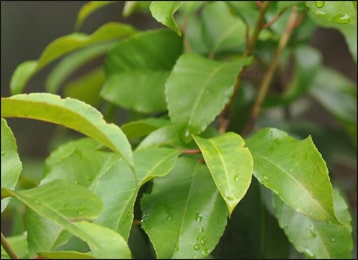This is a close-up photograph of a collection of light green, elongated leaves that are somewhat skinnier than typical tree leaves. The leaves appear healthy, with water droplets glistening on their surfaces, suggesting recent rain or deliberate watering. The main stems attaching the leaves to the plant exhibit shades of red and green, while the central veins of the leaves are a light yellow. Despite the image being heavily focused on the leaves, it also features a blurred background filled with more foliage, giving the impression of an outdoor setting though no other distinct details are visible. The overall sharpness is concentrated on the foreground leaves, which stand out crisply against the more obscure and dark green backdrop.